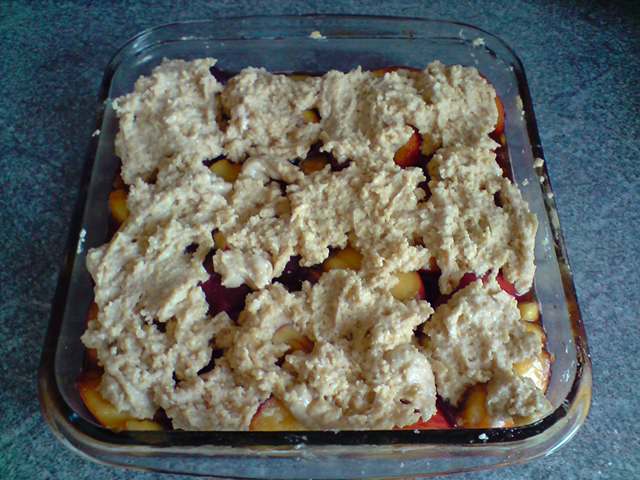The rectangular image is a detailed, close-up photograph of an 8x8-inch clear glass Pyrex baking dish. It is set on a blue marbled countertop, which might be vinyl. Inside the dish, sliced fruit pieces, either apples or peaches with red peels still on, are neatly layered on the bottom. These slices are cut into tiny pieces, likely prepared for baking. Over the fruit, a cream-colored paste of dough is spooned over, resembling the consistency of cream cheese or tuna salad, though it's evidently a kind of dough meant for a cobbler. The unbaked dish is ready and prepared to go into the oven, with some of the dough slightly spilling over the dish's edges.